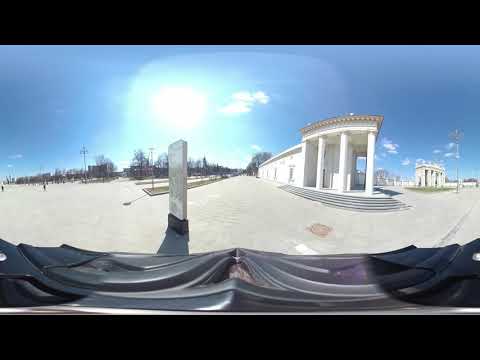This image, captured with a fisheye lens outdoors on a clear day, showcases a vibrant city scene bathed in the bright sunlight of a blue sky with a few diffusing white clouds. Central to the image is a prominent white building on the right side, distinguished by its flat roof and three white pillars, with a small staircase leading to a sprawling, light green sidewalk area. In the middle of this open space stands a rectangular glass plaque or board with a black base. The far right of the image features another white monument-like building with a patch of grass beside it. The horizon is dotted with bare trees, hinting at cold weather, possibly winter, and interspersed with a few distant buildings. The image also includes some light poles seamlessly integrated into the scene. Horizontally across the top and bottom are black strips, possibly a result of the fisheye lens or an added filter, contributing to the curved appearance of the photograph.